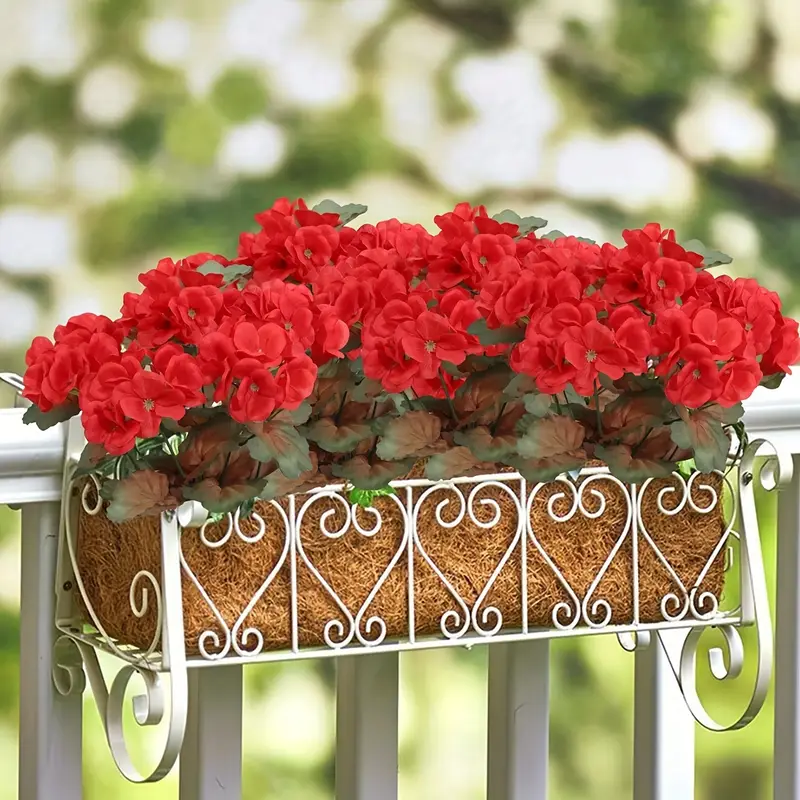The image showcases a close-up of a decorative white wrought iron flower box hanging on a white porch railing. The flower box is intricately designed with metal swirls, forming heart shapes on the front and curved arch patterns on the sides. The container within the metal frame appears to be made of natural straw or a hay-like material, suggesting it might be biodegradable. This rectangular pot houses vibrant red flowers, possibly roses, though their exact type is uncertain. Beneath the flowers, lush green leaves add to the vivid contrast of colors. The background fades into a creamy, blurred bokeh composed of green and white hues, indicating a sunny day with light reflecting off distant foliage. The overall scene evokes a sense of tranquility with its harmonious blend of colors and light.